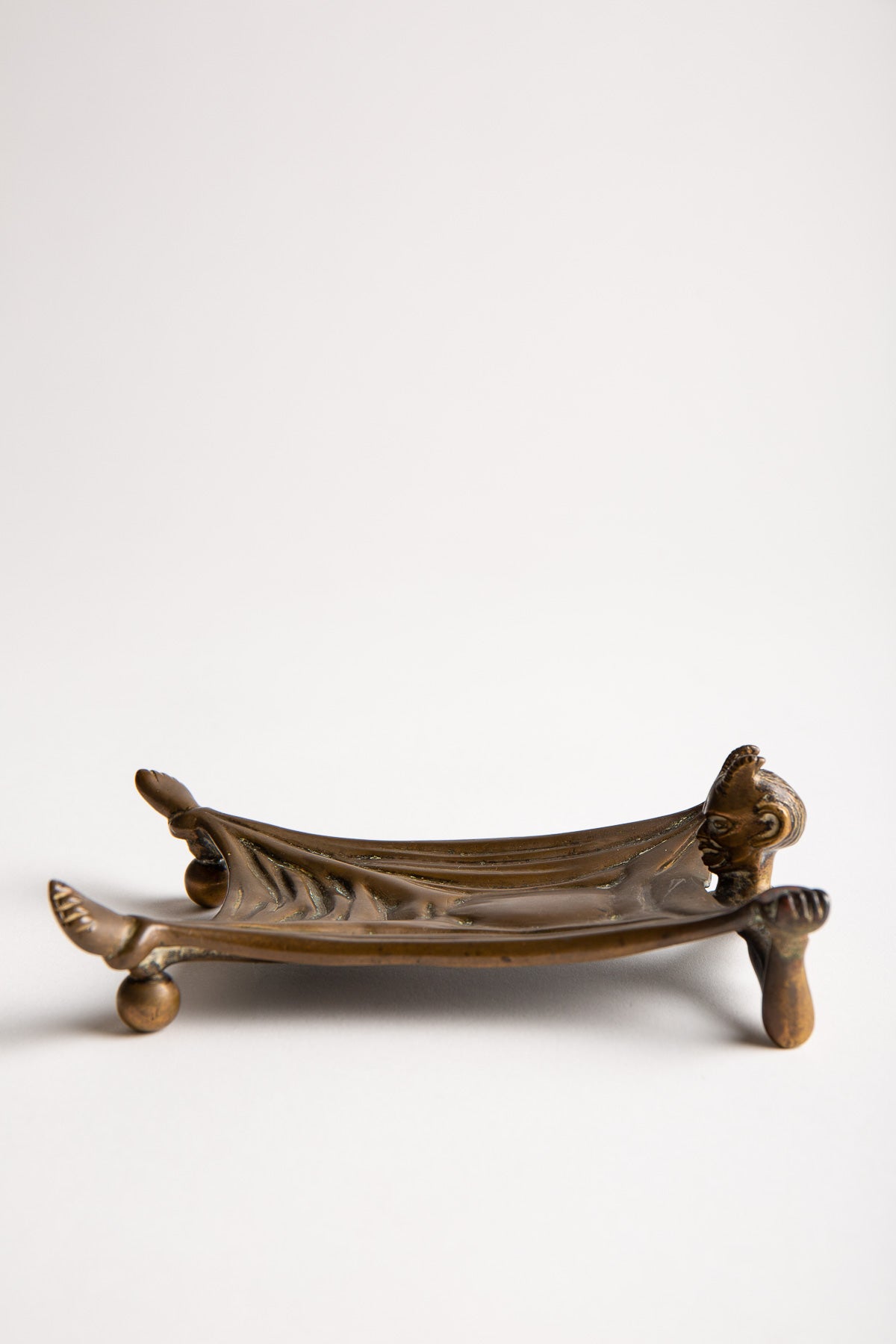In the image, we see a detailed bronze or metallic sculpture resembling a small, stylized piece of furniture placed against a plain white background. The sculpture is situated slightly below the center of the frame, with the shadow of the object distinctly cast underneath it. The figure features a person's head on the right side, along with their hands and legs positioned at different points on the object, creating an intricate, concave structure. The sculpture's design includes two upward-facing, horn-like elements at the front, which complement round balls at the feet forming the front supports. The back legs of the sculpture appear like bent elbows resting on the white surface. This unique piece resembles an old, carefully crafted bowl or tray, with the person's limbs intricately integrated into its design, giving off an impression of the figure lying stretched out with limbs tied, contributing to its artistic and somewhat enigmatic appeal.